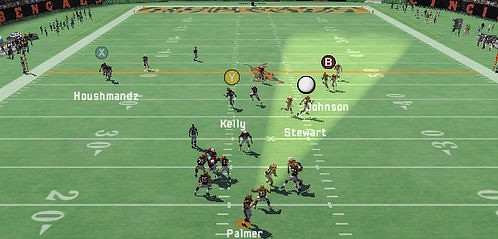Screenshot from a video game simulating an American football match, featuring the Cincinnati Bengals lining up against their opponent. The action is focused between the 20 and 50-yard lines, with players positioned and ready for the next play. Intriguingly, a lone player stands anomalously beyond the 50-yard line, appearing near the unconventional 60-yard marker. Adding a fantastical twist, a dragon is depicted descending onto the field, creating an unexpected and whimsical disruption to the typical football scene.